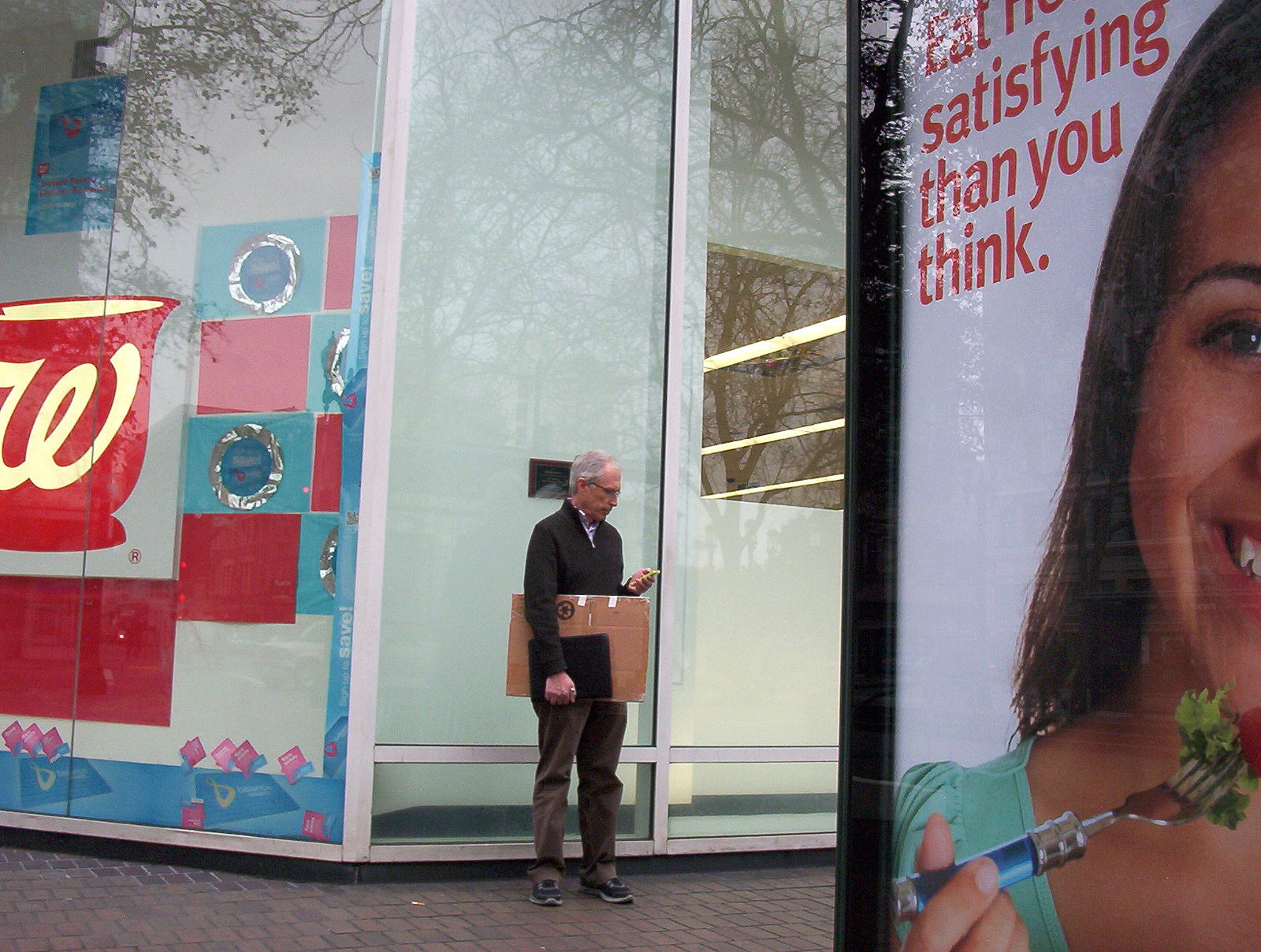An elderly gentleman, with gray hair and glasses, stands on the sidewalk next to a tall glass building. He is dressed in a black sweater, brown pants, and blue shoes. Under his arm, he carries a cardboard box that looks like it might contain a black laptop or briefcase. He is engrossed in his phone. To his left, there are signs on the building that suggest it could be a pharmacy, and you also see a coffee cup icon with a W on the glass window, along with images of silver circles and colored squares in pink, red, and blue. Reflections of trees are visible in the building's glass windows. To his right, there is an image of half a woman's face with black hair, tan skin, and a bite of salad on a blue fork. She is wearing a teal dress, and the advertisement includes the text "eating satisfying than you think." The photo is taken from a position next to this advertisement on the sidewalk.